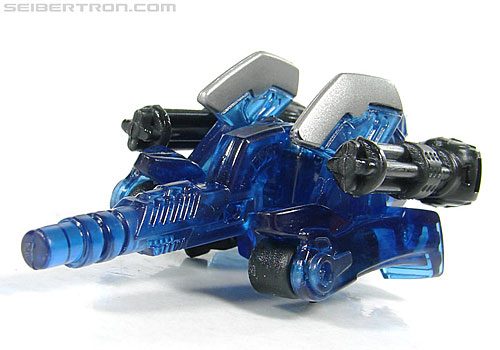In the upper left corner of the image, in light gray font, the text reads "Cybertron.com." The central object in the image appears to be a translucent blue plastic toy, resembling a futuristic device or spaceship. The toy has several distinct features: on the sides, it has two large, gun-like protrusions that are black and shaped like missiles. The upper portion of the toy includes curved pieces that are silver and somewhat wing-like. Additionally, there are gray bolt-like elements extending from the sides, possibly imitating lasers. At the base of the toy, it has black wheels which contribute to its lifted appearance, almost like the front of an army tank. Overall, the object has a high-tech, robotic aesthetic consistent with a toy from a sci-fi universe.